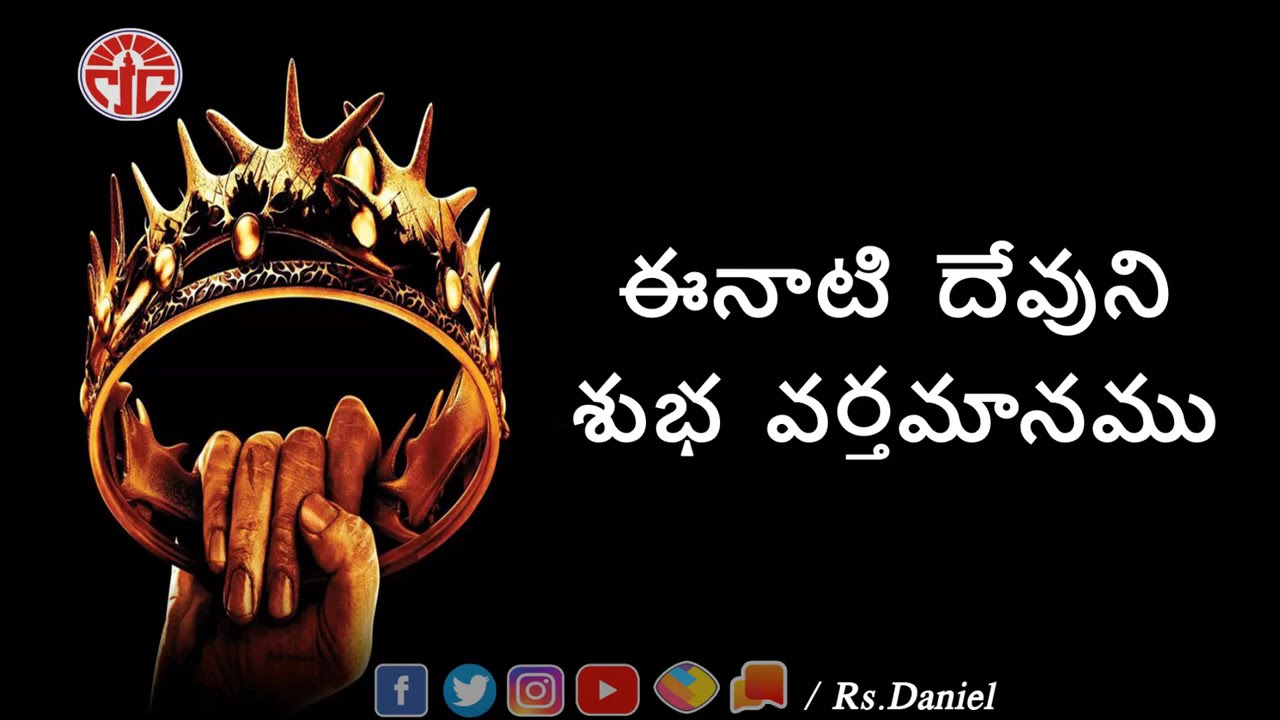This image appears to be a meticulously designed graphic with a black rectangular background. Dominating the left side of the image, there's a detailed hand-drawn crown with bony spikes, seemingly fashioned from tarnished gold and adorned with gold gems. A hand is shown holding this intricate crown aloft. In the upper left corner, there's a white circular icon featuring a complex red design within it. To the right side of the crown, there's a curvy, curly script written in white, which appears to be in Arabic or Hindi, though the exact language is unclear. At the very bottom of the screenshot, spanning across the lower edge, are several social media icons: Facebook, Twitter, Instagram, YouTube, and two additional icons—one resembling a diamond shape with a colorful design and the other comprising overlapping orange and red banners. Adjacent to these icons, the text "RS.Daniel" is displayed prominently.